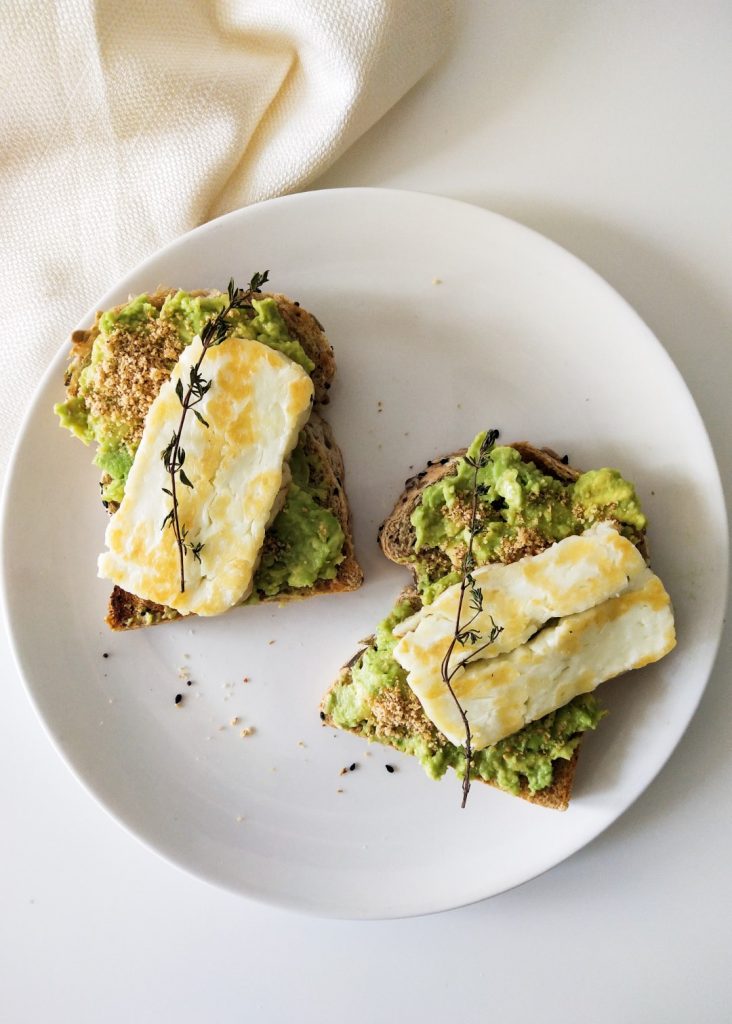This tall rectangular aerial photograph features a breakfast meal meticulously arranged on a pristine white ceramic plate, set against a matching white surface. A casually folded white woven napkin rests in the top left corner, adding a touch of homely charm. The central focus of the dish includes two slices of light brown toast, sprinkled with dark black seeds; one slice positioned towards the top left and the other diagonally beneath it to the right. Generously spread atop the toast is a vibrant green mashed avocado. Crowning the avocado is a somewhat rectangular piece of cheese, exhibiting a delightful browning from being lightly cooked, resulting in appetizing yellowish-brown patches. To finish, an elegant black herb branch is artfully placed across each piece, lending an element of sophisticated garnish reminiscent of a chef's touch.